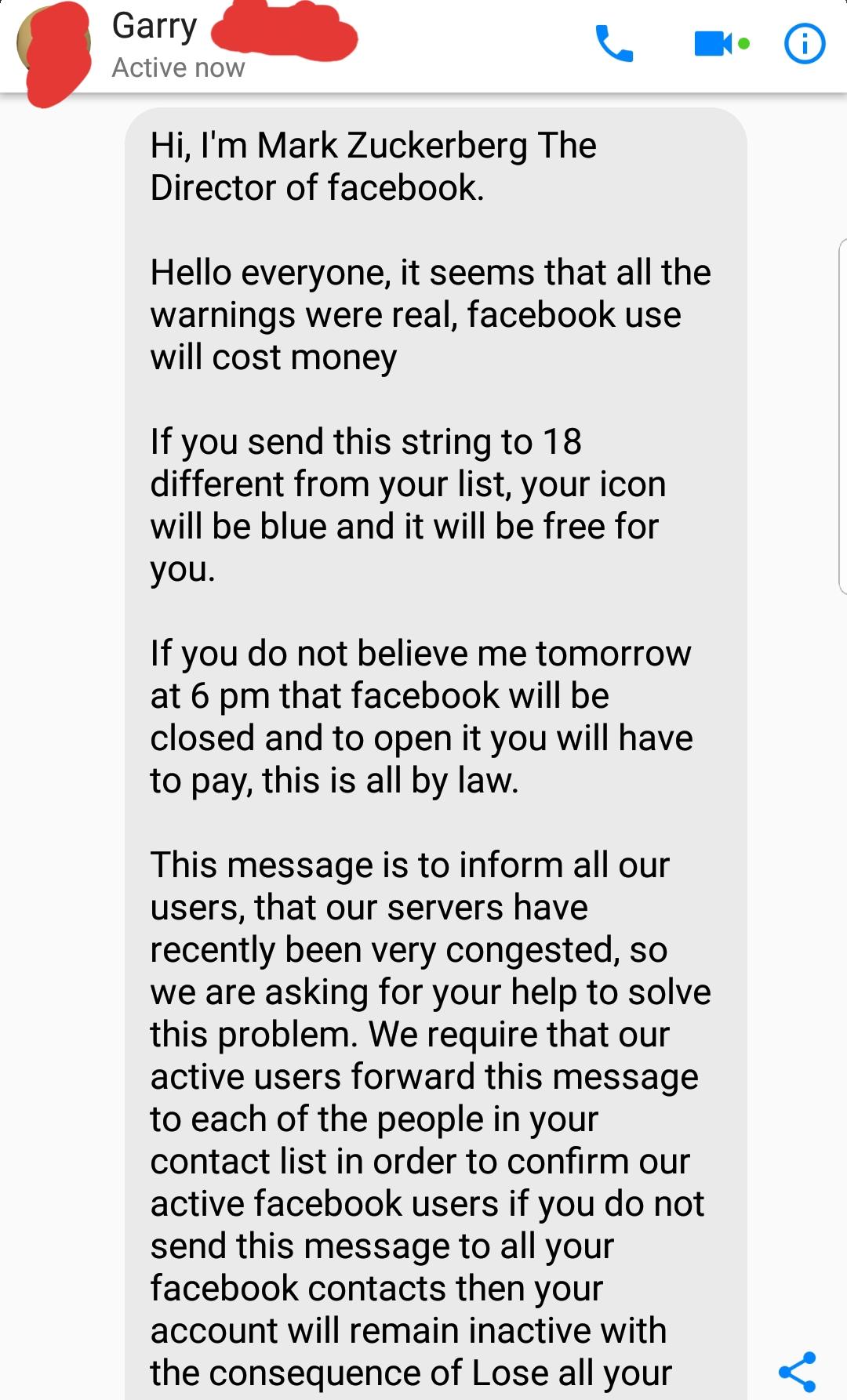The image is a screenshot of a Facebook message, seemingly from a person named Gary—identified by a blurred-out profile picture and a last name scribbled out in red ink. Gary is marked as "active now." The message, which appears to be a suspicious chain letter, starts with the text: "Hi, I'm Mark Zuckerberg, the director of Facebook. Hello everyone, it seems that all the warnings were real. Facebook use will cost money. If you send this string to 18 different from your list, your icon will be blue and it will be free for you. If you do not believe me, tomorrow at 6 p.m. that Facebook will be closed, and to open it, you will have to pay. This is all by law. This message is to inform all our users that our servers have recently been very congested, so we are asking for your help to solve this problem. We require that our active users forward this message to each of the people in your contact list in order to confirm our active Facebook users. If you do not send this message to all your Facebook contacts, then your account will remain inactive with the consequences of lose all your..." and the message cuts off mid-sentence. The message header also includes icons for phone, video call, and information, all in blue, with a gray text box and a blue share button located at the bottom right.